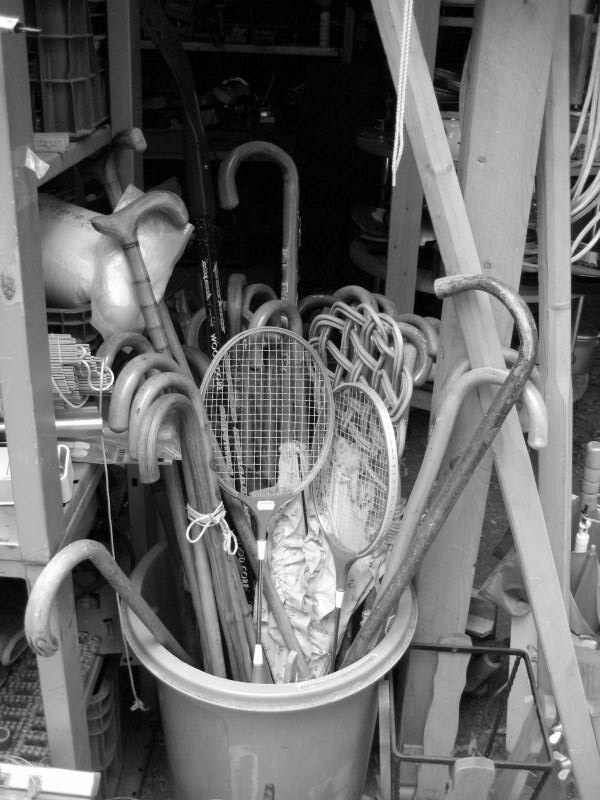The black-and-white photograph captures the interior of a cluttered garage. Central to the image is a large plastic bucket brimming with approximately 10 walking canes and a couple of vintage tennis rackets, possibly accompanied by a hockey stick and a bamboo cane. Surrounding the bucket are tall, slender wooden planks stacked vertically to the right. To the left, shelves crowded with various knick-knacks and additional walking canes are visible, adding to the disarray. An empty wire basket organizer is also noticeable among the items. The background transitions into a stark black shadow, hinting at more items beyond the reach of the light, emphasizing the garage’s densely packed nature.